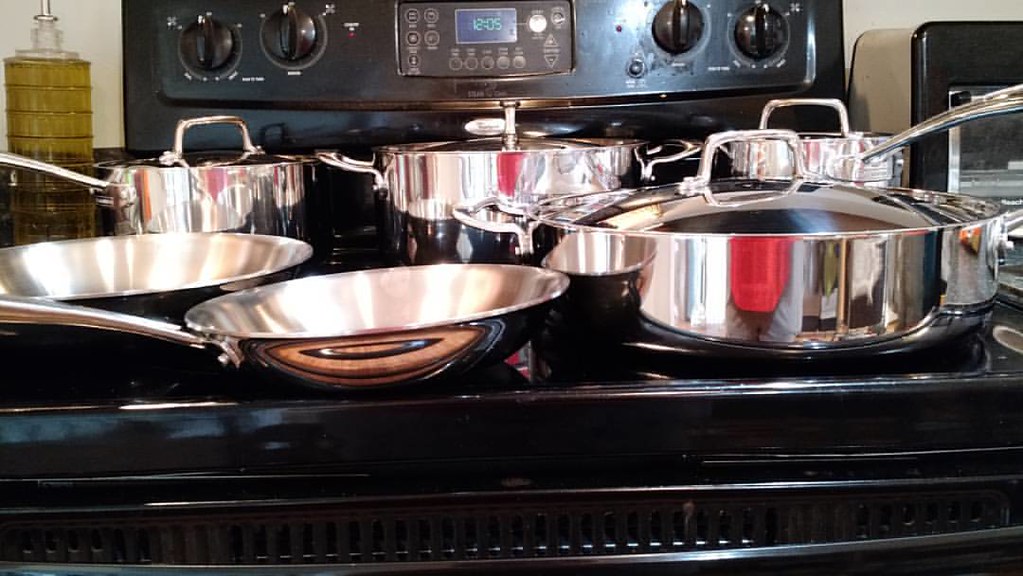This high-quality, color photograph, taken indoors in landscape mode, showcases a black stovetop adorned with brand-new, reflective silver cookware. The stove features four black dials—two on the left and two on the right—and a central control panel with an LCD screen displaying the time as 12:05 in green numbers against a black background. On the stove's three back burners sit three shiny metal pans with lids, while the front burners hold a large deep frying pan with a clear glass lid, another similar pan behind it, and two omelet pans on the left. Each piece of cookware boasts silver or chrome color with reflective surfaces, accentuating their new, unused state. To the right edge of the image, a glimpse of another black cooking surface or stove is visible but not fully in the shot. Additionally, a clear glass bottle is seen in the top left corner of the stove. The stovetop does not appear to be in use, as no flames are visible beneath the burners.